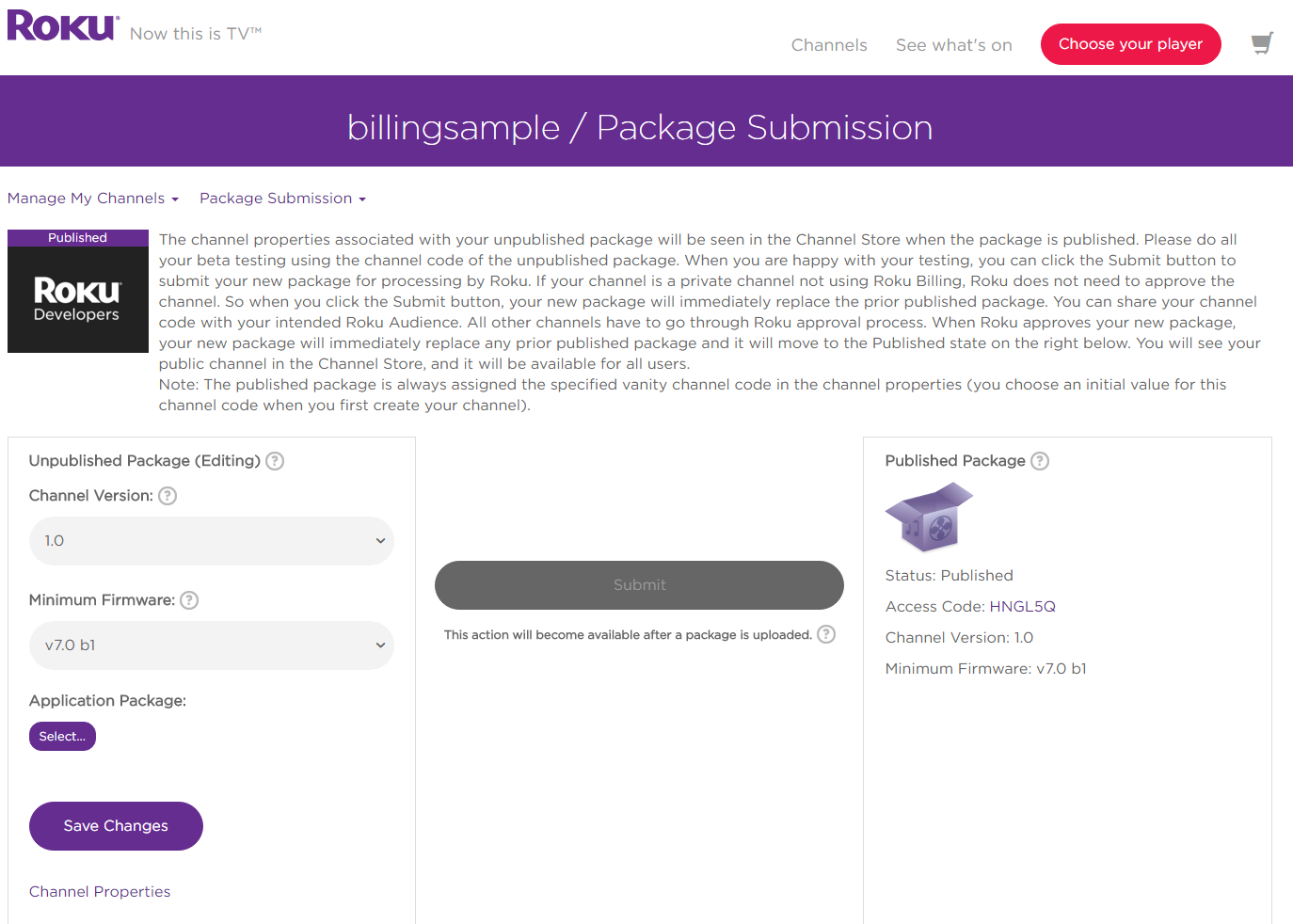**Detailed Caption:**

The image features a Roku interface with a layered, detailed layout. At the top left, the text "Roku" is prominently displayed in blue, followed by the tagline "Now this is TV" written in black. Adjacent to this on the top right are several toggles or tabs labeled "Channels," "See What's On," and "Choose Your Player." These elements are set against a red background, creating a striking contrast.

Below this red section, the background shifts to a deep purple hue, showcasing the text "Billing Sample or Package Submission." Beneath this section, the text continues on a white background, providing detailed instructions and information in a clear format. 

The white-text section provides comprehensive guidance for Roku developers, explaining the process for managing channel packages. It instructs users to conduct beta testing using the channel code of the unpublished package. Once satisfied with the testing, developers can click the "Submit" button to proceed with package submission. It explains the differences in processes for private channels not using Roku billing versus other channels that require Roku's approval.

Additionally, the right panel details the status of the published package, including the "Access Code: hngl5q," "Channel Version: 1.0," and the minimum firmware version required, "v7.0." On the left, tabs provide options for editing the "Unpublished Package" and display the current "Application Package" details, with changes savable as needed.

In the center, instructions indicate that the "Submit" action will become available once a package is uploaded. Overall, the interface is neatly organized and user-friendly, guiding developers through the channel submission process with clarity and precision.